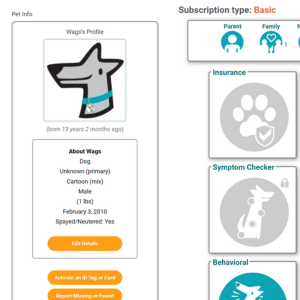**Caption:**

The image depicts a form screen designed for entering pet information against a white background. On the left side, the header "Pet Info" is displayed, while the right side shows "Subscription Type: Basic." The left panel is bordered in gray and appears cut-off at the bottom, indicating continuation beyond the visible area.

At the center of the form, there is a white box with a blue outline featuring a cartoon dog's head. This section is titled "Wag's Profile," with a subtext in gray stating "Born 13 years, 2 months ago."

Below this, there is a vertically oriented rectangular box detailing the dog's profile. It reads:
- "About Wag's Dog:
  - Unknown primary (Cartoon Mix)
  - Male
  - 1 pound 
  - Born February 3rd, 2010 
  - Spayed/Neutered: Yes"

An orange button with the text "Edit Details" is positioned beneath these details. Following this are two additional orange buttons, "Activate on ID Tag or Card" and "Support: Report Missing or Found."

On the right side of the form, there are square buttons labeled "Parents," "Family," "Insurance," "Symptom Check," and "Behavioral."